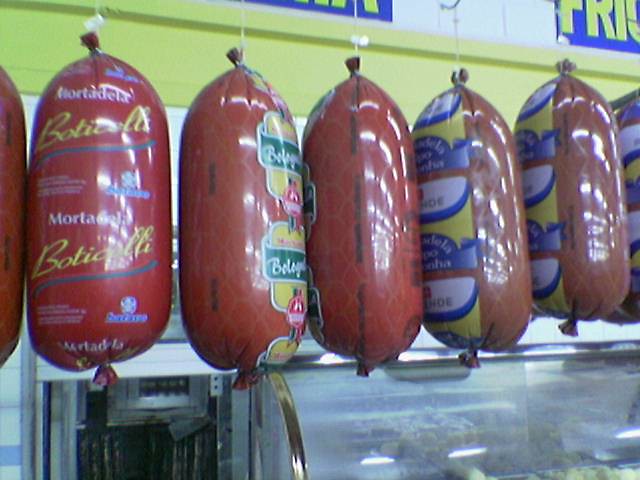The image captures a vibrant scene in a supermarket's meat department, likely a deli. Suspended from the ceiling, a row of large, plump mortadella sausages hang in plastic casings, ranging in color from reddish-brown to red. The plastic casings are clear, showcasing the sausages' robust appearance, almost as if they are about to burst. Each sausage is secured with a tie on each end and adorned with various labels – some yellow with blue and white accents, others yellow with green, and one prominently displaying "mortadella Botticelli" in yellow letters with blue trim. In the background to the right, there is a rounded glass meat case with a white counter, and some indistinct items can be seen at the bottom right, possibly other food products. Above this, the wall is white with a large blue sign featuring yellow writing, beneath which runs a long yellow strip. The overall scene is brightly lit, with reflections from overhead lights visible on the shiny surfaces of the sausages.